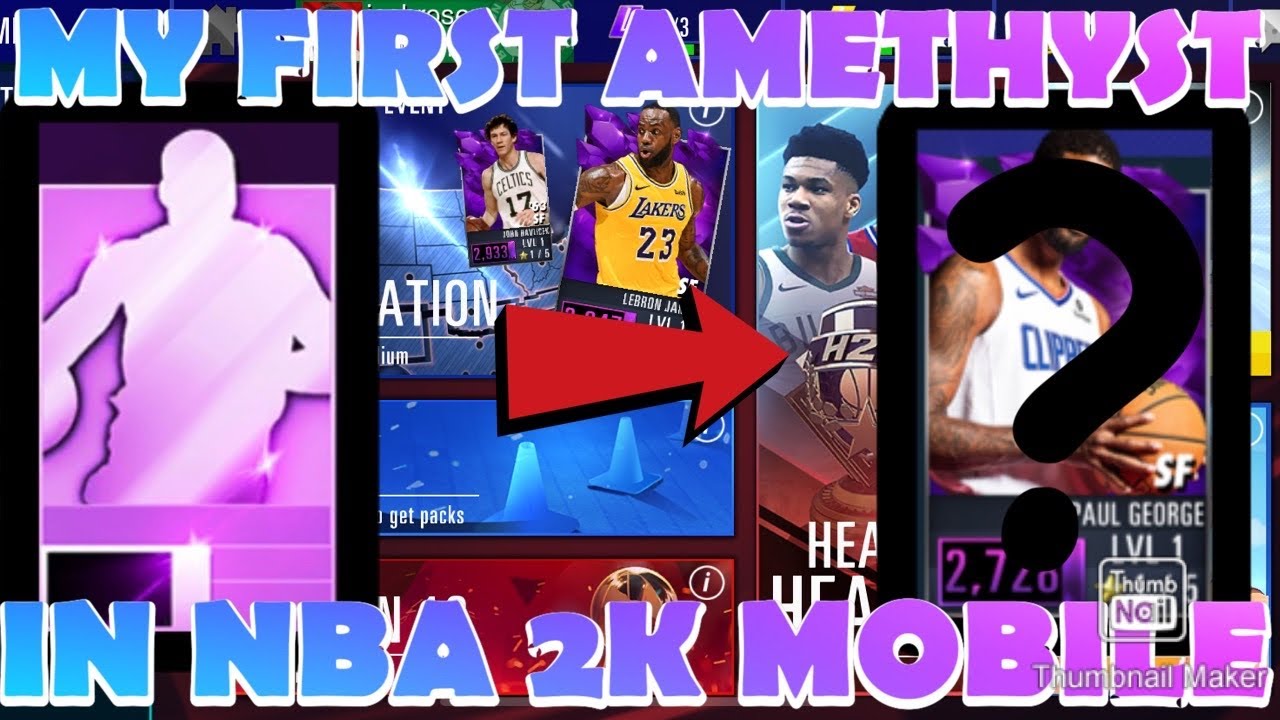This is a detailed description of a screenshot from a web page, taken on a desktop, laptop, tablet, or smartphone, showcasing NBA players. At the top of the screenshot, the text reads "My First Amethyst," with "My" and "First" in predominantly blue text, transitioning into purple for the letters "RST." The word "Amethyst" is gradient-colored, starting from purple and fading into pink at the end.

At the bottom of the screenshot, the text "NBA 2K Mobile" appears. "NBA" is mostly blue, but the letters "B" and "A" transition into purple. "2K" is fully purple, and "Mobile" transitions from purple to pink, with "M" and "O" in purple, and "B" mostly purple that slightly fades to pink, before transitioning fully to pink.

On the left-hand side, there is a pink rectangle with sparkles, featuring the silhouette of an NBA player. On the right-hand side, another rectangle displays an African American NBA player with short hair wearing a white Clippers jersey with blue lettering. Below the player, the text "2.72" is partially covered by a question mark drawn in black. The text "Paul George" is also present, though partly obscured by the question mark. Below his name, it reads "Level One" in gray text.

In the center of the image is LeBron James, flanked by two other individuals whose names are cut off from the view on the left and right-hand sides.